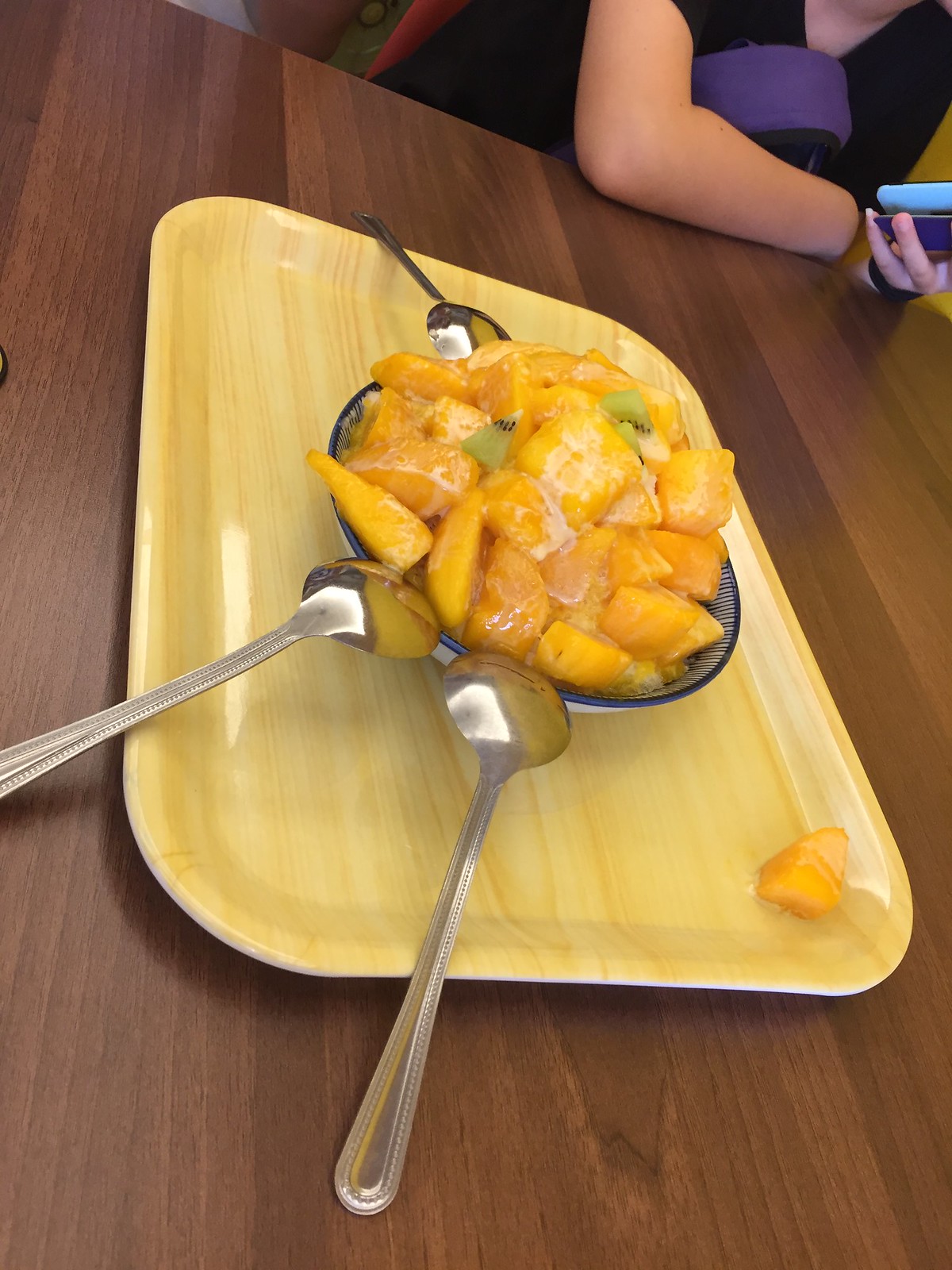In this detailed color photograph, a blue and white bowl filled with a vibrant fruit salad, featuring slices of kiwi, peaches, cantaloupe, and possibly oranges or mangoes, is placed on a pale yellow cafeteria tray. This tray rests on a faux wood grain tabletop. Three silver spoons are propped face down on the edges of the bowl, leaning outward. A single piece of the orange fruit has strayed to the bottom right corner of the tray. In the background, the arm of a young woman clad in a black t-shirt is visible as she leans her elbow on the table. She holds a pale blue cell phone in one hand, and a purple object is tucked in the crook of her other arm.